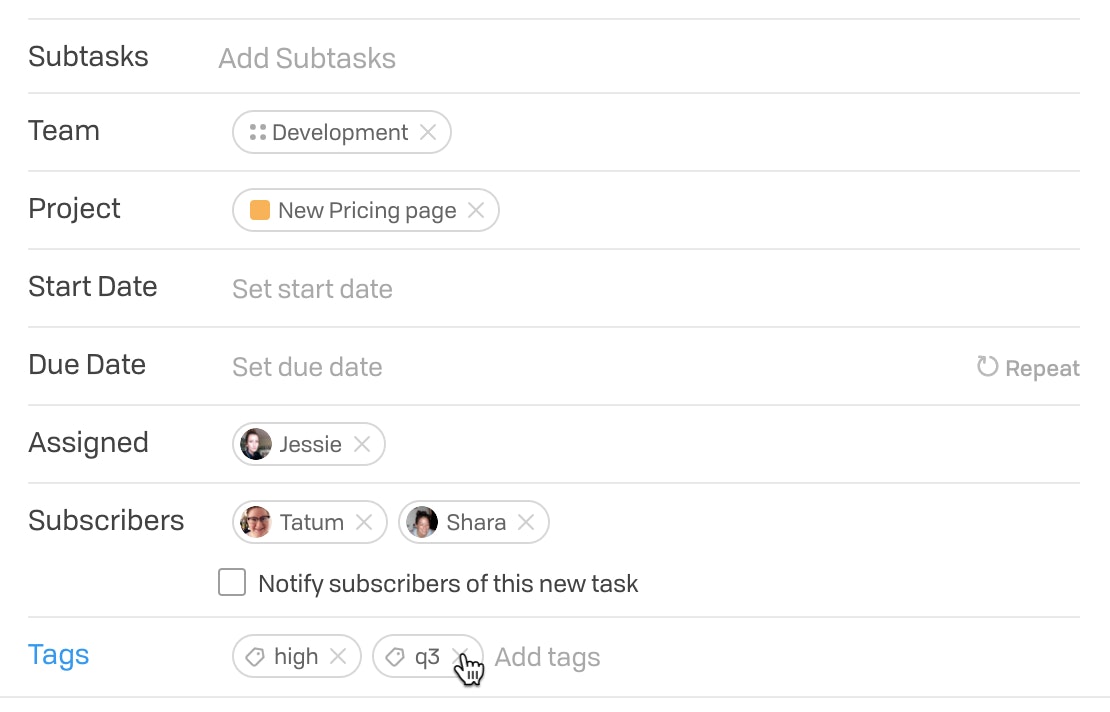The image is a screenshot from a computer, displaying a task management interface against a white background, organized into different rows.

- **Top Row:** The first row is labeled "Subtasks." To the right, in gray text, it says "Add Subtasks."
- **Second Row:** The next row is labeled "Team." To the right of this, there is an oval-shaped button labeled "Development," followed by an 'X' button.
- **Third Row:** The row below says "Project," with "New Pricing Page" written to its right, accompanied by another 'X' button.
- **Fourth and Fifth Rows:** The subsequent row is labeled "Start Date," and to its right, it says "Set Start Date." Directly below this is "Due Date," with "Set Due Date" next to it.
- **Sixth Row:** The next row is labeled "Assigned." Adjacent to this is an oval shape containing a picture of a female, labeled "Jessie."
- **Seventh Row:** Underneath "Assigned" is "Subscribers." To the right of this, there are two oval-shaped circles, one labeled "Tatum" and the other "Shara," each containing a picture of a female.
- **Eighth Row:** Below the subscribers, there is a checkbox labeled "Notify Subscribers of this new task."
- **Ninth Row:** The final option is "Tags," presented in blue. To its right, there are bubbles labeled "Hi" and "Q3," followed by "Add Tags." A finger is pointing at the 'X' next to the "Q3" bubble.

This screenshot provides a detailed overview of various task attributes and management options available in the interface.